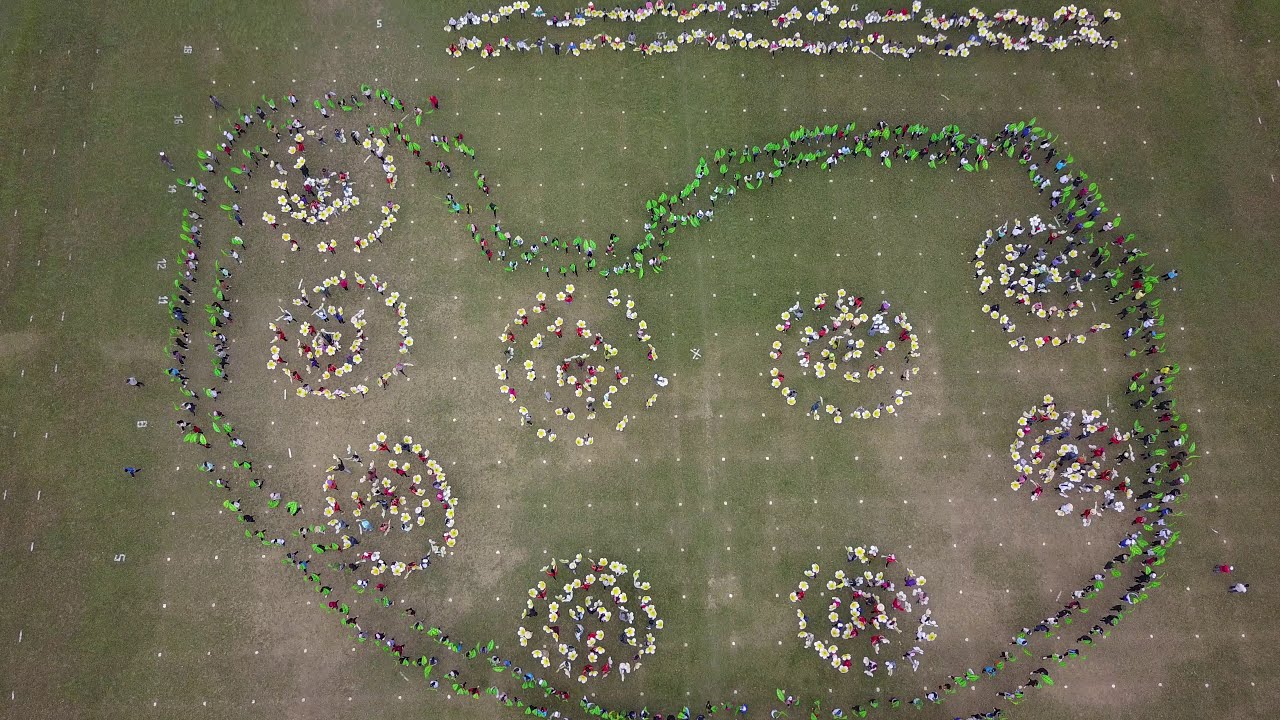This landscape-oriented, color photograph, captured from high above by a drone, presents a detailed and intricate scene on a grass field segmented into a grid by tiny white squares. The image showcases a large formation of people arranged in a kidney-shaped design. The outer border of this shape features two rows of individuals holding green flags. Within this border, the composition reveals a pattern of spirals and circles formed by groups of people predominantly holding white flags. Towards the top of the image, two additional horizontal lines of closely grouped people in white attire can be observed. The arrangement includes varied colors such as green, yellow, red, pink, black, and brown accents, creating a vibrant and organized visual spectacle against the natural outdoor setting.